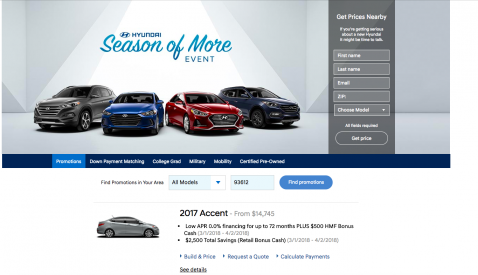The screenshot showcases an advertisement for the "Hyundai Season of More Event." Dominating the image is a photograph featuring four vehicles: a gray SUV on the far left, followed by a blue coupe, a red sedan, and a blue-gray SUV on the far right. The background of the image is predominantly gray and white, with the event title displayed prominently in blue text.

To the right side of the vehicle lineup, a gray column features a call to action in white text: "Get Prices Nearby." Below this, there is a form to input personal details, including first name, last name, email, zip code, desired model, and a button to "Get Price."

Immediately beneath the photo of the vehicles, a dark blue bar is labeled with various promotional categories: "Promotions, Down Payment Matching, College Grad, Military, Mobility, Certified Pre-Owned." Directly below this bar, the text prompts users to "find stores in your area," "all models," and provides a field to enter a zip code, shown here as "93813."

The bottom section of the ad highlights specific deals, including a 2017 Hyundai Accent priced from $14,745. The offer includes low APR financing at 0.2% for up to 72 months, a $500 HMF bonus cash, $2,500 total savings in retail bonus cash, and options to "Build & Price," "Request a Quote," "Calculate Payments," and "See Details."